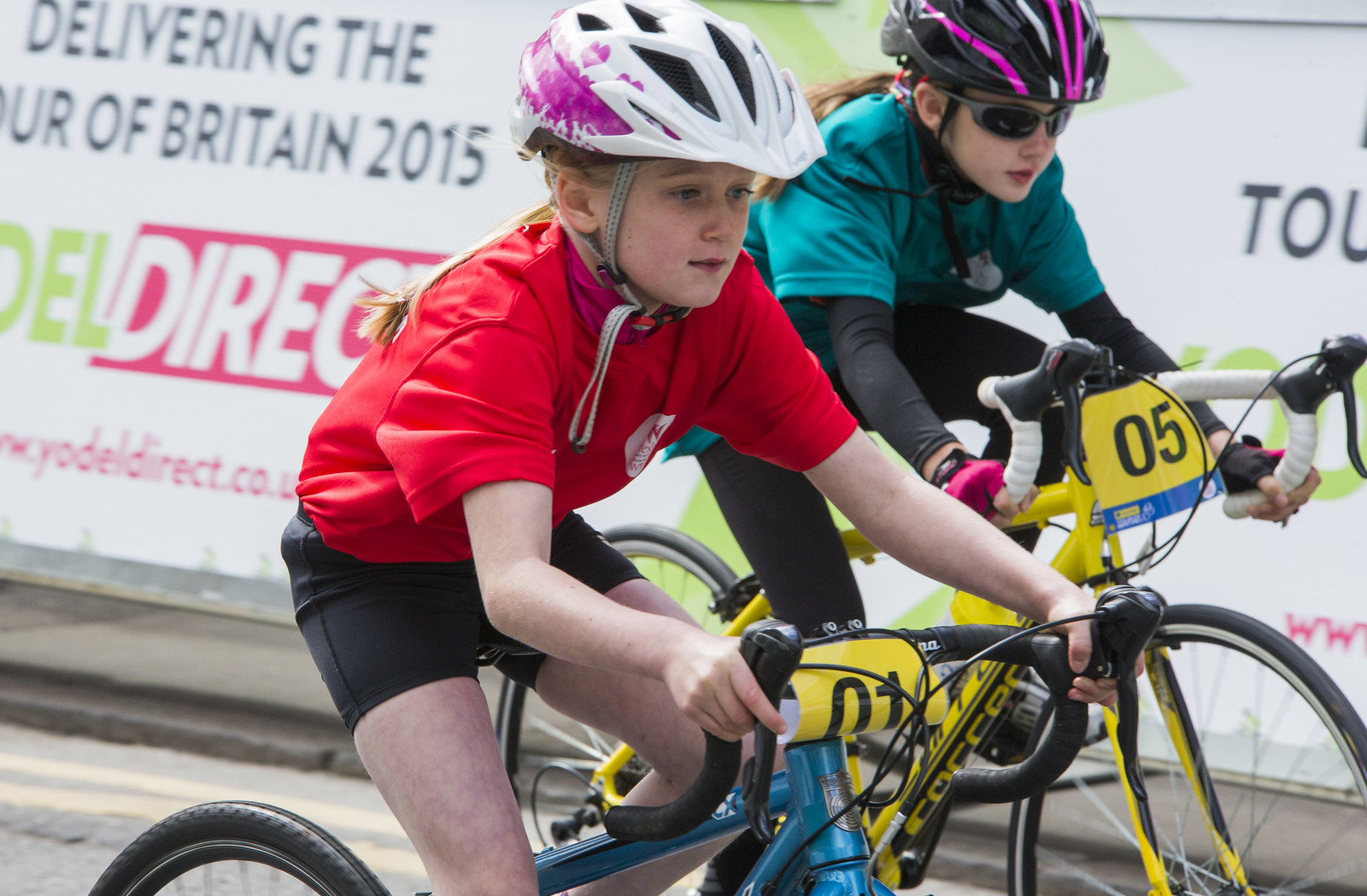This image captures a close-up of two girls, likely children or young teenagers, participating in an organized bike race. They are riding side-by-side on sleek, road-style bicycles, suggesting a competitive event. Both riders are wearing helmets and have long hair tied in ponytails.

The girl closest to the camera, distinguished by her blonde hair and white helmet with pink trim at the base, is wearing a red t-shirt and black bike shorts. She rides a light blue bike marked with the number "01" on a black card mounted on the front, and her bike features blue handlebars. She appears very focused on the race.

Next to her, the second girl sports a black helmet with pink and white stripes, framed sunglasses with gray lenses, a turquoise t-shirt over a long-sleeved black shirt, and black leggings. She is riding a yellow bike, with the number "05" displayed on a yellow card. Her handlebars are strikingly wrapped in white tape.

Both girls are pedaling intently as they pass by a banner that reads "Delivering the Tour of Britain 2015" in black letters at the top left. The banner also includes sponsor logos and a website URL in pink and green letters. Despite their differing attire, the girls seem evenly matched as they race side by side, embodying the spirited competition typical of youth sports.